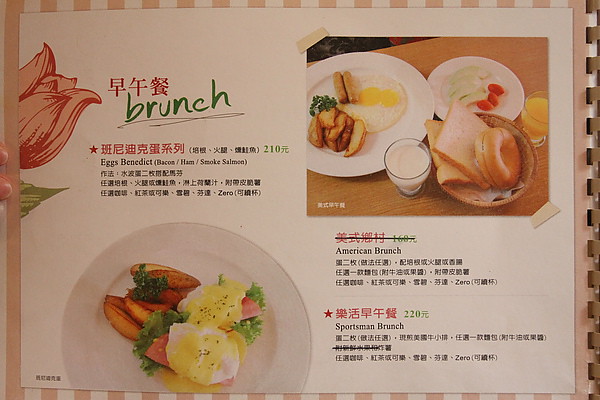The photograph captures a restaurant menu printed on a light-colored piece of paper, featuring a background of pink and white stripes. The menu is neatly bound with a spiral holder. At the top, a tulip image complements the word "BRUNCH" written prominently. The menu includes characters in a foreign language alongside English dish names. Below, it lists options such as "EGGS BENEDICT" with choices of bacon, ham, or smoked salmon, as well as "AMERICAN BRUNCH" and "SPORTSMAN BRUNCH." Accompanying the text are vivid pictures of delectable food plates. One image showcases potato wedges garnished with parsley, ham topped with eggs, and a generous layer of yellow sauce. Another picture displays a hearty plate featuring two fried eggs, two sausage links, crispy fried potatoes, a refreshing glass of milk, and a basket filled with a bagel and slices of bread.